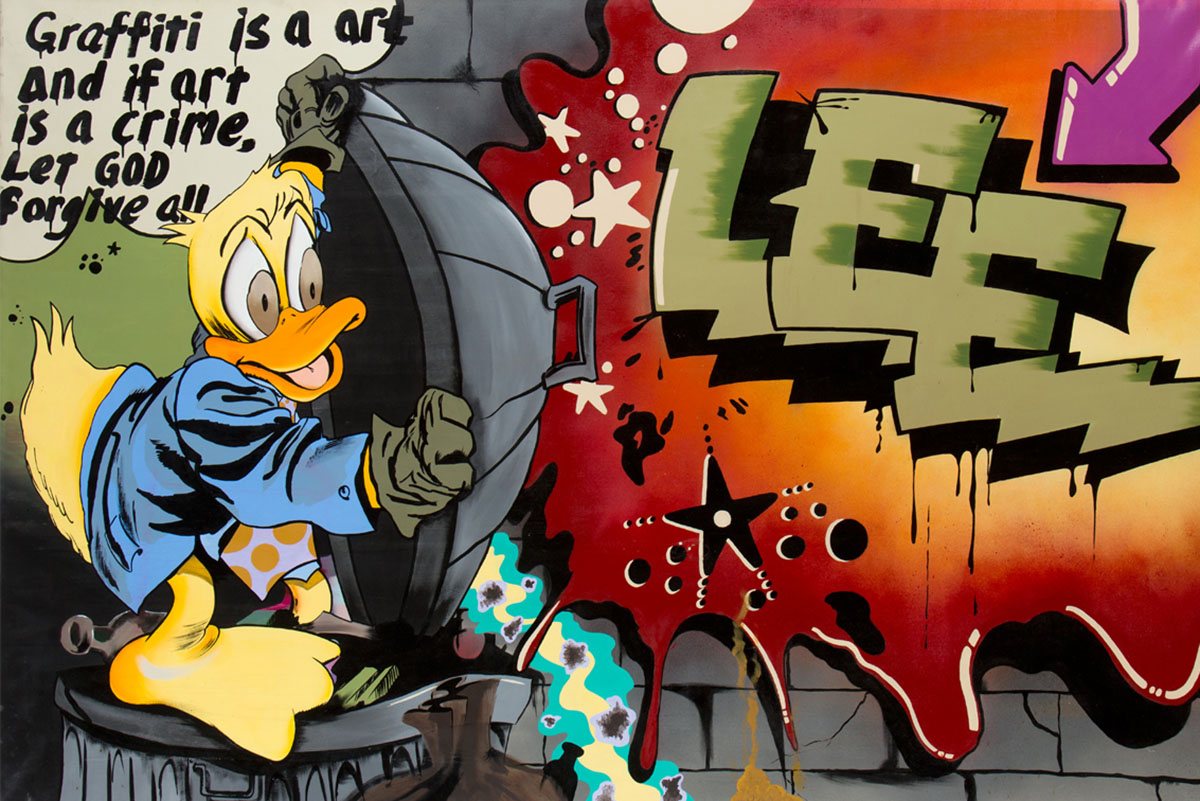The poster is a full-color, horizontally-oriented illustration that depicts a cartoon duck reminiscent of Donald Duck, standing on a gray garbage can on the left-hand side. The duck is yellow with an orange beak, wide eyes, and wears a blue jacket, polka dot tie, and green gloves. He holds the garbage can lid in his right hand, seemingly engaged in the act of painting graffiti. To the right, in vibrant graffiti style, the letters "L-E-E" are written in green against a gray wall, highlighted by a dripping red and orange circle that looks like a text bubble. Above the letters, a purple arrow points to the graffitied name, accompanied by black and white stars and round orbs. In the upper left-hand corner of the poster, the text reads, "Graffiti is an art, and if art is a crime, let God forgive all," encapsulating a modern, edgy theme. Additional blue and white squiggles to the left of the graffiti resemble something spilling from the trash can, adding to the chaotic, street-art atmosphere of the scene.